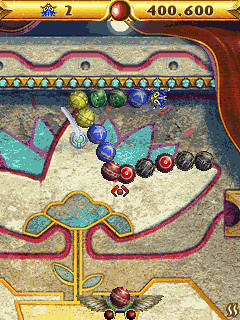In this vertically oriented rectangular image, we see a screenshot from the video game "Zoom". The scene is set in an area with an Egyptian theme, characterized by its use of golds, browns, blues, reds, and yellows. The gameplay features a stream of multicolored beads or balls traveling along pathways, resembling an elaborate assembly line. At the top right corner of the image, the current score is displayed as "400,600" in red text against a gold background. To the left of the score, the number "2" is visible, likely indicating the player's current level or stage.